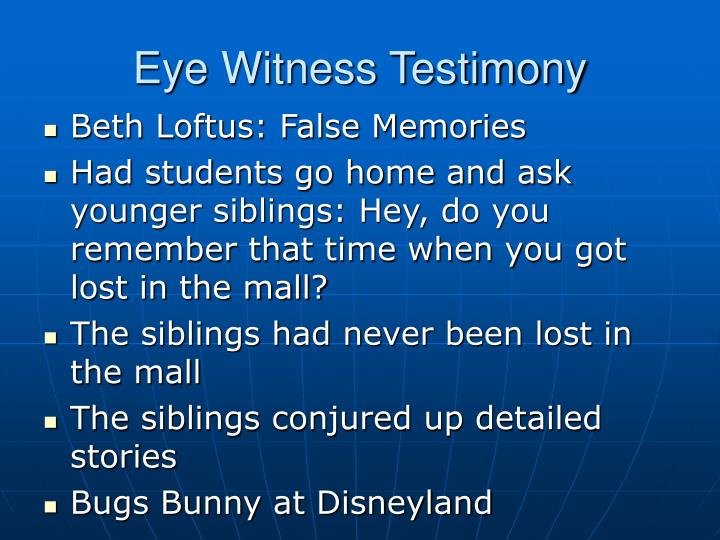The image features a slide with a gradient blue background transitioning from light blue at the top to dark blue at the bottom, overlaid with a grid pattern reminiscent of latitude and longitude lines. At the top of the slide, "Eyewitness Testimony" is prominently displayed in white text. Below this title, there are five bullet points, each marked with white bullet boxes, listing key concepts related to false memories:

1. Beth Loftus: False memories
2. Had students go home and ask younger siblings: "Hey, do you remember that time when you got lost in the mall?"
3. The siblings had never been lost in the mall.
4. The siblings conjured up detailed stories.
5. Bugs Bunny at Disneyland

The overall layout and design suggest an educational or legal context, with a clean and clear presentation focused on the phenomena studied by Beth Loftus regarding the creation of false memories. The colors utilized include varying shades of blue, white, and hints of black, adding to the polished and professional appearance of the slide.